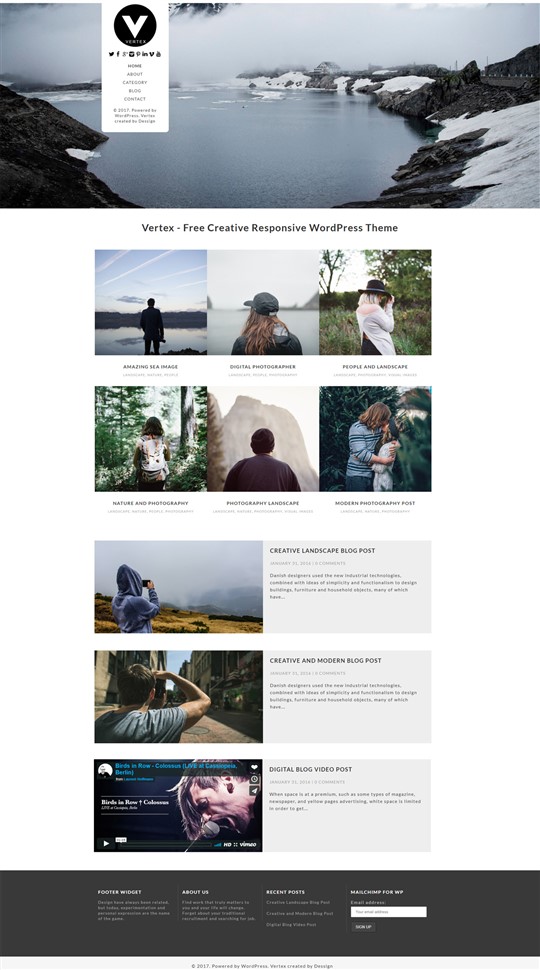A series of ten horizontally oriented photographs, displayed in a sequence of seven frames, portrays various scenic and nature-inspired shots, all with the overarching theme of exploration and solitude. Each frame highlights moments of serene beauty, fostering a calming aesthetic. Despite the small size of the images making it difficult to decipher details, the predominant elements are discernible.

At the top, the first image depicts an ocean bordered by land with icy formations dotting the shoreline, likely part of a frozen landscape. Below this image, the text reads: "Vertex - Free Creative Responsive WordPress Theme." The company name, starting with the letter 'V,' is printed in very small text and is challenging to read.

The second segment comprises three images: 
1. A man silhouetted against a colorful horizon, possibly at sunset, staring contemplatively into the distance.
2. A woman sharing a similar stance, facing away from the camera towards the vast ocean and overlying mountains.
3. Another woman, clad in a jacket and hat, capturing a photograph in a dense forest or a national park enveloped by trees.

The third segment includes three more pictures, maintaining the theme of back-facing subjects immersed in majestic scenery such as mountains and national parks, reinforcing the sense of connection with nature’s grandeur.

In the final segment of the sequence, the last three photographs feature:
1. A person photographing a landscape shrouded in dense fog.
2. A perspective over a deep canyon.
3. An indiscernible image, which, while unclear, aligns with the series' overarching motif of nature and exploration.

Overall, these ten images, spread across seven frames, appear to be part of a visual presentation for a WordPress theme aimed at showcasing the beauty of nature and human reflection within it.